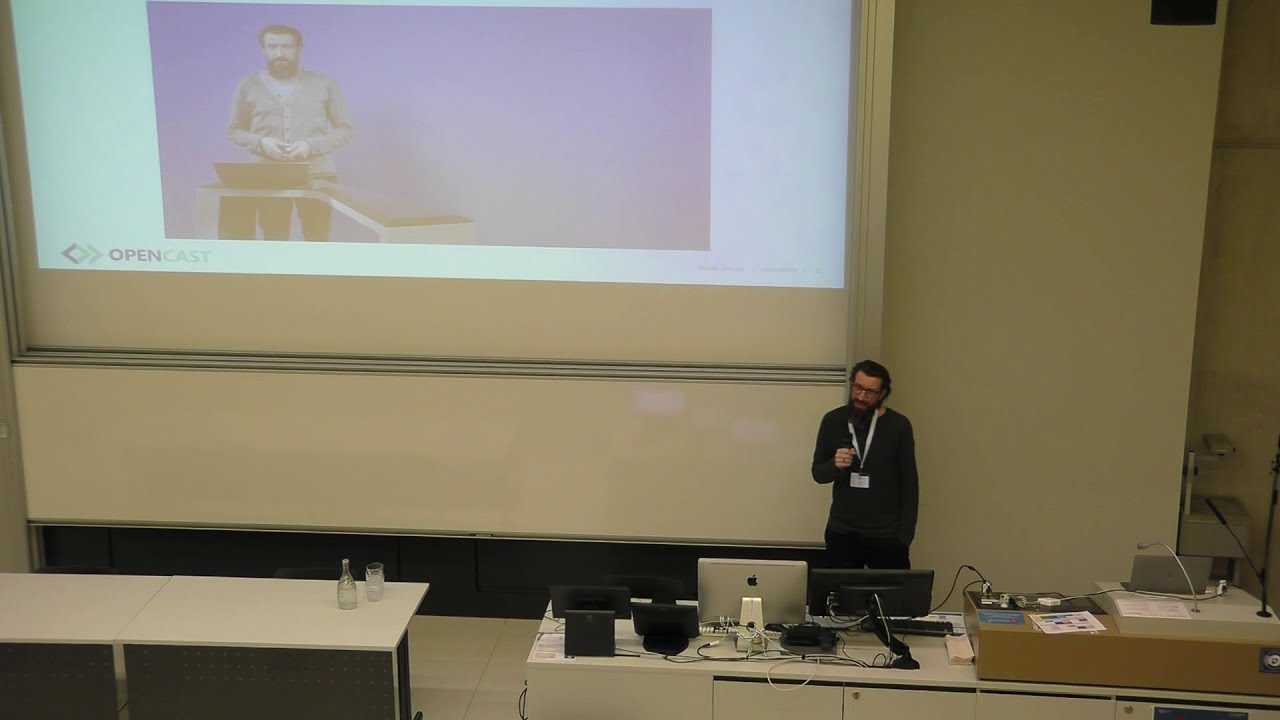The image appears to be a screen capture from a university lecture, shot from a high-angle perspective typical of stadium-style seating in a large classroom. It features a middle-aged man, likely a professor, wearing a long-sleeved black shirt, glasses, and a white lanyard with a name tag. He has a beard and mustache and stands behind a desk equipped with two computer monitors, various wires, and papers. There is another desk to his left with a white tabletop holding a bottle and a drinking glass. The room is dimly lit, emphasizing the large projector screen behind him, which displays a projection of the same man, labeled with the text "Open Cast," possibly indicating the topic of the lecture or a previous recording.